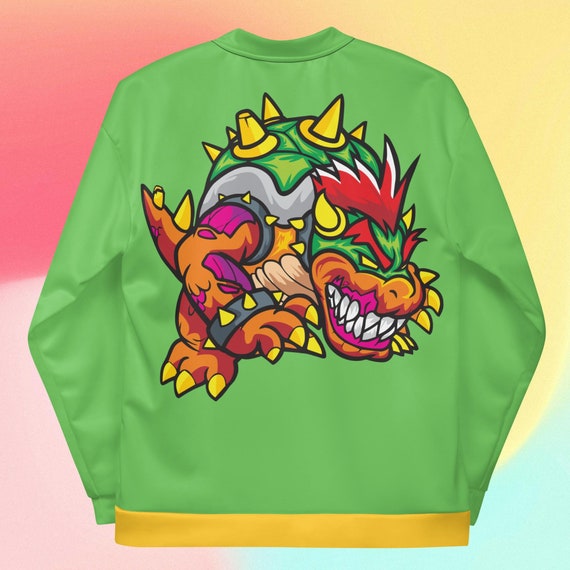The image depicts a digitally enhanced photograph of a lime green long sleeve sweatshirt, likely designed for online retail platforms like Amazon. The background is a multicolored gradient with pastel hues: pink fading to peach and yellow in the upper corners, light mint green in the lower right, and pale pink in the lower left. The sweatshirt features a bold, colorful cartoon dragon character reminiscent of Bowser from the Mario Brothers video game. The dragon has a green head with yellow horns and fiery red eyebrows. Its orange face frames a mouth with magenta gums and sharp white teeth. The creature has a green turtle shell adorned with yellow spikes and a beige underbelly. Its arms are orange with purple accents, and it has an orange tail. The bottom border of the sweatshirt is accentuated by a yellow stripe running across it.